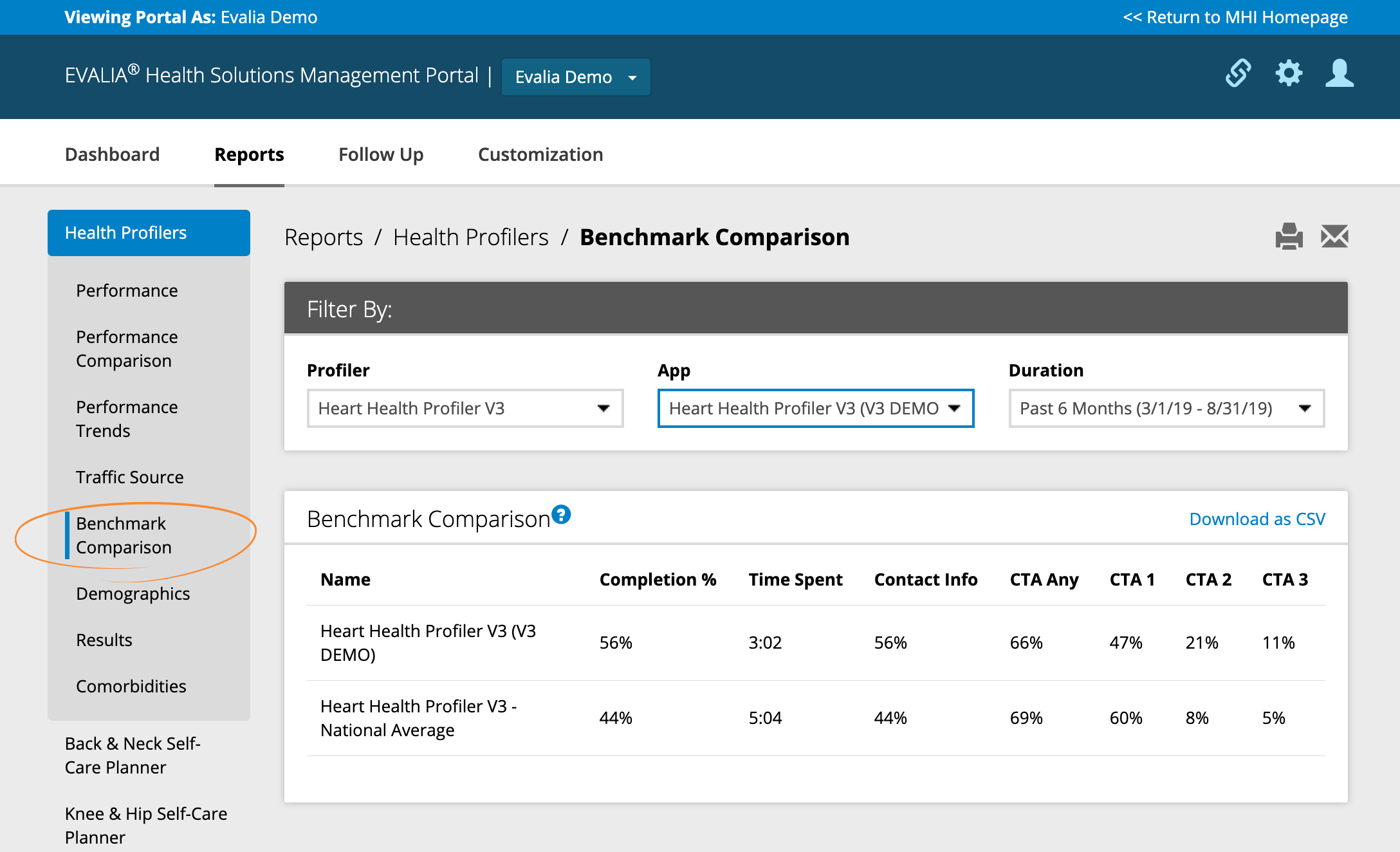Featured here is the Ivalia Health Solutions Management Portal's homepage. The top section of the page displays a two-toned bar, with an ink blue color transitioning into a dark navy blue. At the very top, the text reads "Viewing Portal: Ivalia Demo" on the left, and "Return to MHI Homepage" on the right. Below this bar, the header prominently announces "Ivalia Health Solutions Management Portal" with a drop-down box that is set to "Ivalia Demo."

Towards the top-right corner, there are icons for copying links, accessing settings, and a user profile. The central section of the page begins with a row of tabs on the left including: Dashboard, Reports, Follow-up, and Customization.

Beneath these tabs is a vertical list of options:
- Health Profilers
- Performance
- Performance Comparison
- Performance Trends
- Track Traffic Source
- Benchmark Comparisons (highlighted with a yellow circle)
- Results
- Demographics
- Back and Neck Self-Care Planner
- Knee and Hip Self-Care Planner
  
In the center of the page, there is a section labeled "Filter By" for sorting through benchmark comparisons.